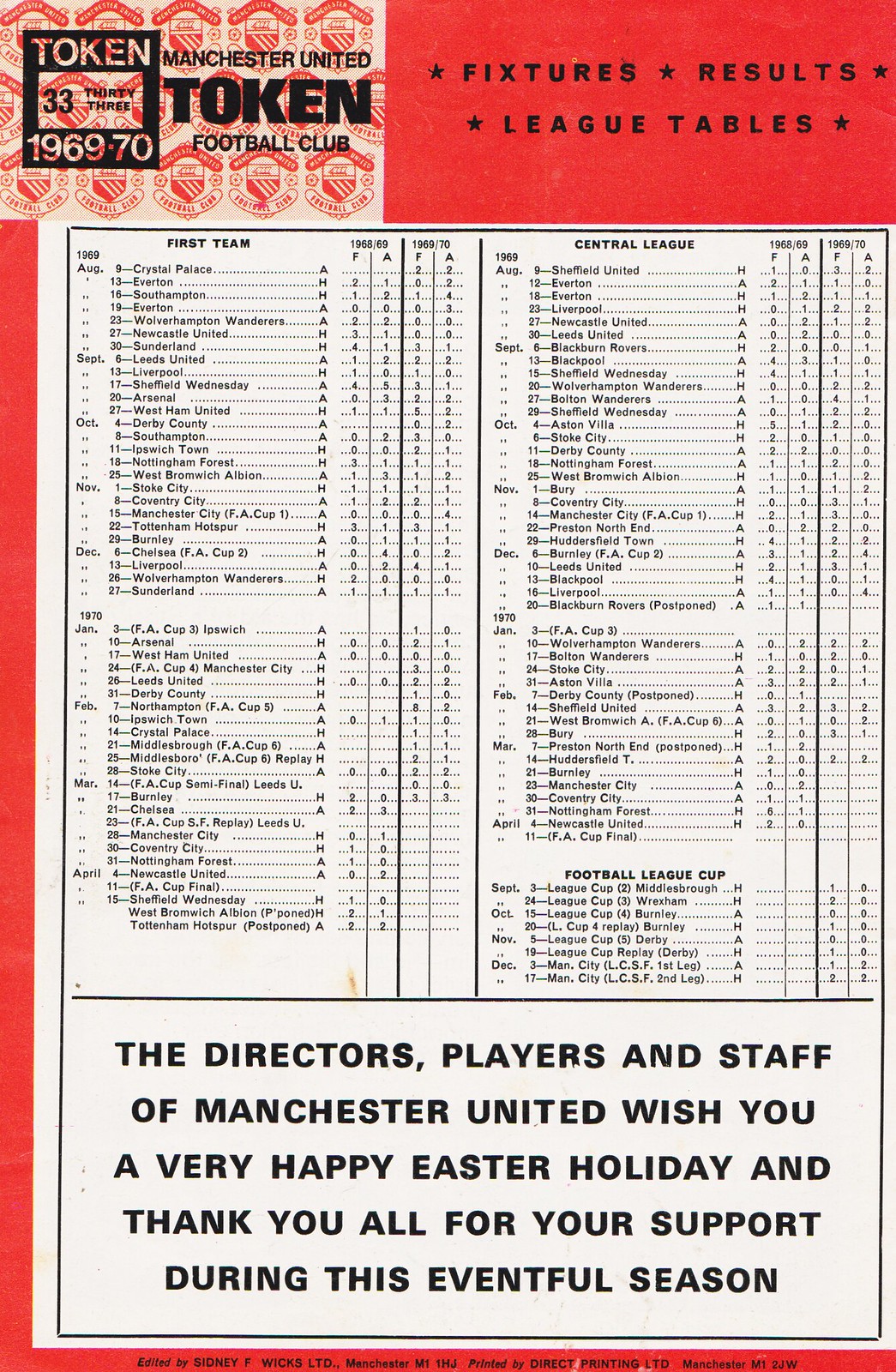This photograph captures a detailed directory for the Manchester United Token Football Club from the 1969-70 season. The overall background is red, with the directory's data presented on a white background with black text. In the upper left corner, the title "Manchester United Token Football Club" is prominently printed in black text on a red background. Adjacent to this, a black square contains the text "Token 33, 1969-70." To the right, a red section headlines with "fixtures, results, league tables" in black letters.

Within the main body of the chart, detailed columns list player names and their associated statistics. On the left side, the "first team" roster is organized by month, presenting a comprehensive view of the team's performance. Correspondingly, the right side features data for the Central League, segmented similarly by month and statistical figures.

At the very bottom, a bold statement in black on a white background extends warm holiday wishes and gratitude: "The directors, players, and staff of Manchester United wish you a very happy Easter holiday and thank you all for your support during this eventful season." This message underscores the collective acknowledgment and appreciation for the fans' support throughout the season.